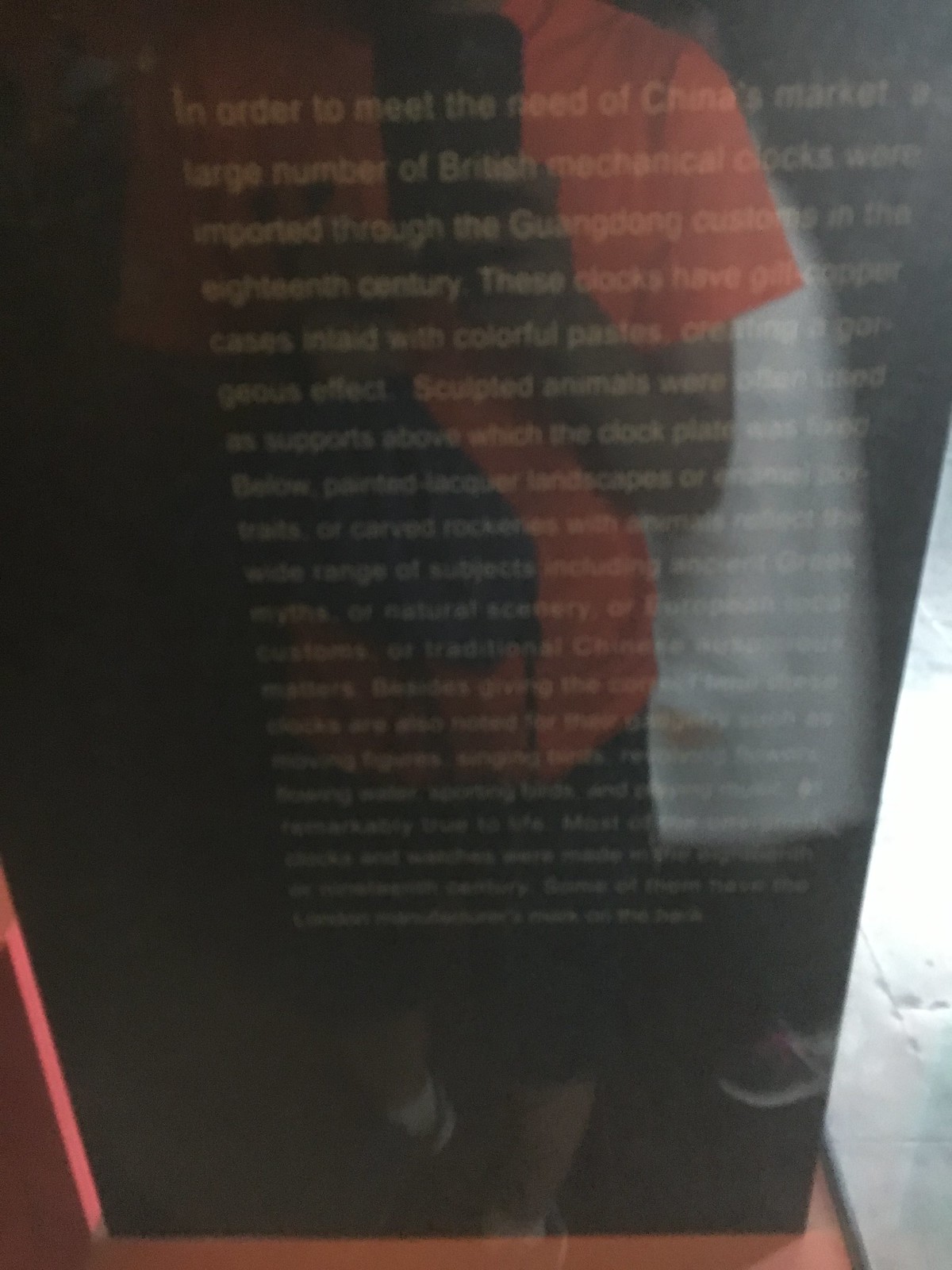The photograph captures a museum plaque encased in glass. The reflection on the glass reveals the photographer, distinguished by an orange t-shirt and partial view of their legs and shoes. The plaque itself contains extensive text, which appears to detail the history and mechanics of clocks used in Chinese markets. The context and setting strongly suggest that the image was taken in a museum exhibit focused on mechanical clocks.